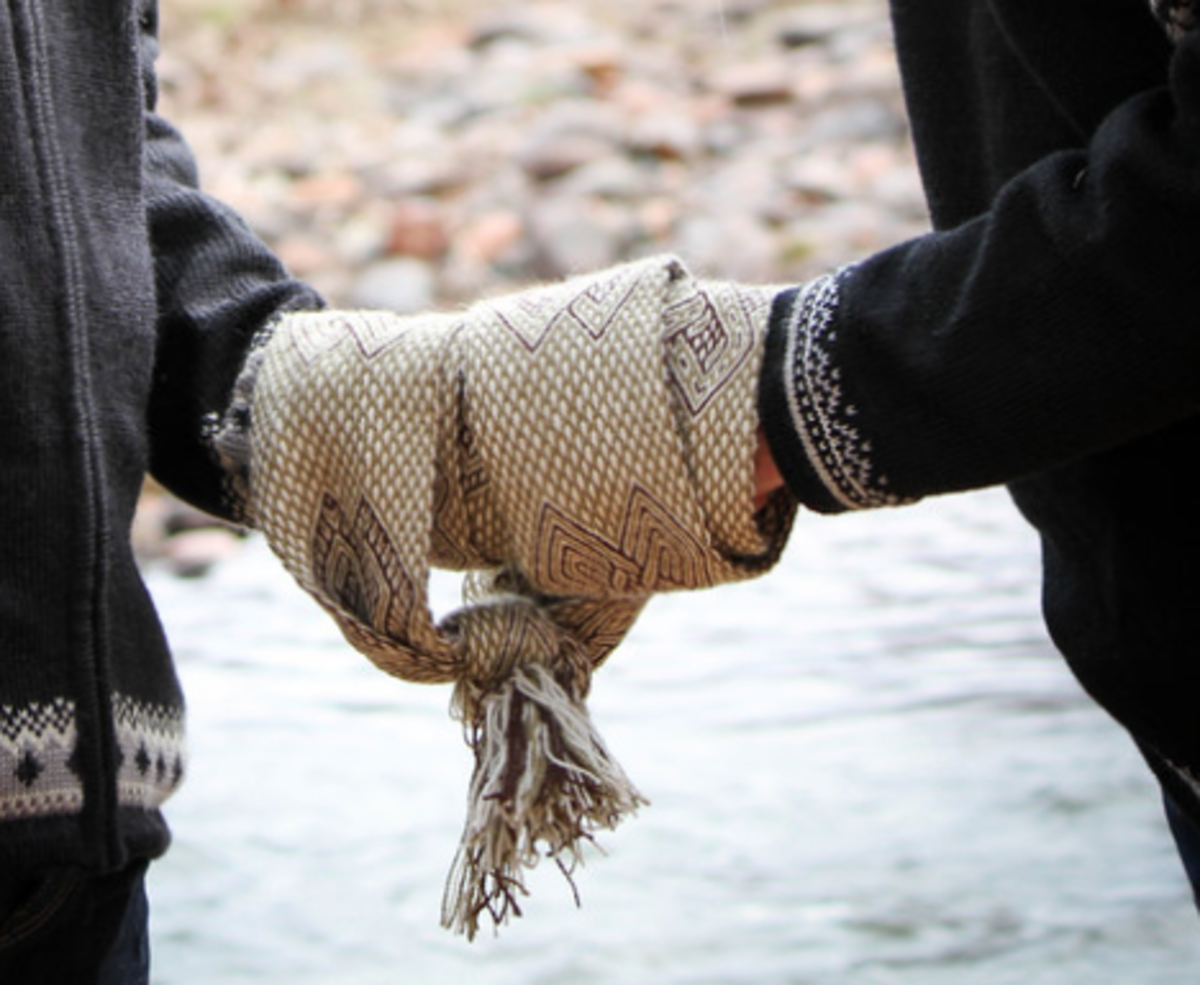The image captures an outdoor scene with a blurred background that vaguely suggests rocks and possibly water. It predominantly features the mid-sections of two individuals facing one another, dressed in sweaters with distinctive white trim. The person on the right wears a black sweater, while the person on the left wears a gray one with some intricate white and gray designs near the bottom. Their arms extend towards each other, with their hands enveloped together by a beige-patterned tapestry. This woven cloth, decorated with triangular and possibly maroon and gold insignia and finishing in frayed tassels, is wrapped around their hands and tied in a knot, evoking a sense of union or ceremonial commitment, possibly a wedding ritual. The general aesthetic and design of the sweaters suggest a Nordic or tribal indigenous influence.